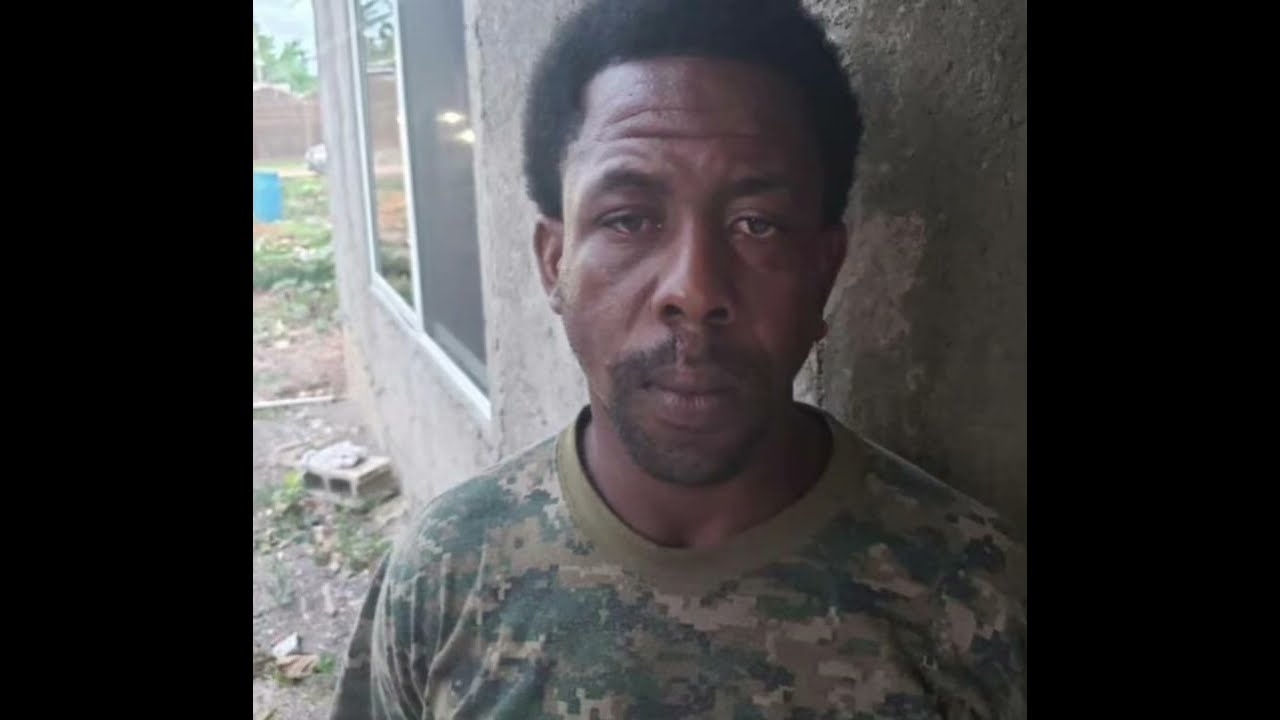The image is a horizontally rectangular photograph with thick black borders on the left and right. Positioned just right of center is an African American man, likely in his 30s or 40s, facing the camera with a neutral expression. He has short black hair, dark eyes, and sports a mustache and a light goatee. The man is wearing a camouflage-patterned t-shirt in various shades of green. He stands outdoors, next to a large concrete building with tan and brown walls. Over his left shoulder, a wall adorned with white-framed windows stretches out, revealing some foliage and a light blue sky in the background. Nearby on the ground, a square white object is visible under the windows, and there's a light blue barrel or structure further back. The ground is predominantly dirt with some vegetation visible to the left.